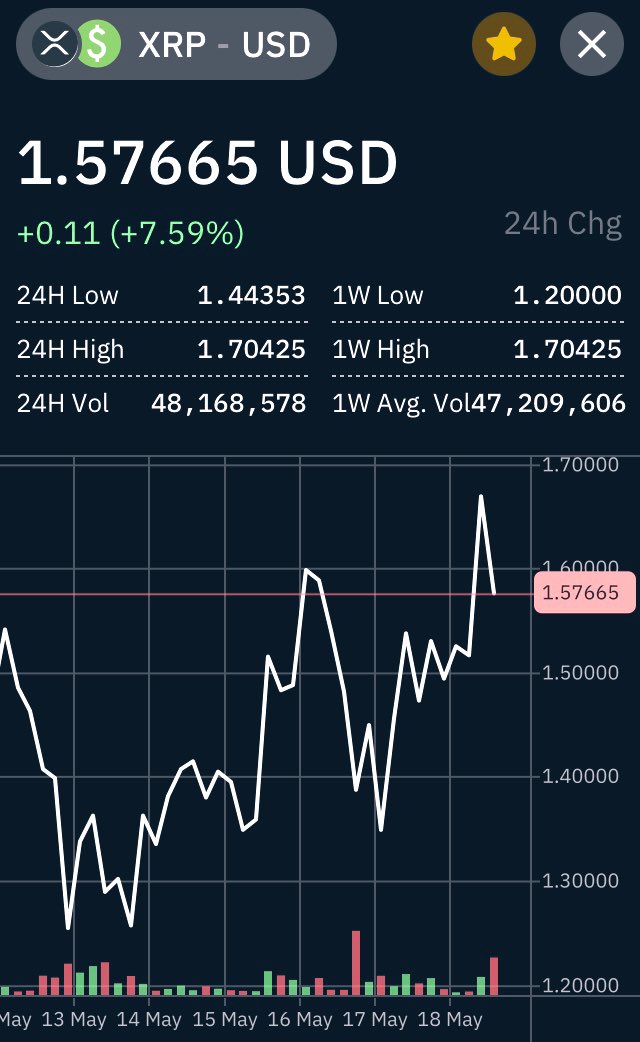The image features a detailed view of a cryptocurrency data page displayed against a black background. In the top left corner, a green circle encloses a white dollar sign, symbolizing currency. Next to this icon, the text "XRP USD" is prominently displayed, indicating the cryptocurrency pair.

In the top right corner, an orange star within a circle is present, signifying a featured or favorite item. Adjacent to it, a dark gray circle contains a white "X", possibly for closing or dismissing an item.

Beneath these icons, the current value of the cryptocurrency is shown as "1.57665 USD". Below this, metrics indicating a 24-hour change are detailed: "plus 0.11, plus 7.59%, 24-hour CHG". Further down, data points about the day's trading range and volume are listed:
- "24H low: 1.44353"
- "24H high: 1.70425"
- "24H vol: 48,168,578"

On the right side, performance over the past week is highlighted with these figures:
- "1W low: 1.200000"
- "1W high: 1.70425"
- "1W average vol: 47,209,606"

Below all this information, a graph provides a visual representation of the cryptocurrency's price movement from May 13 to May 18. The white line on the graph fluctuates between the lowest value of "1.200000" and the highest value of "1.70000". A pink box prominently highlights the number "1.57665", emphasizing the current price.

This detailed summary presents a comprehensive overview of the cryptocurrency's performance and key statistics over specified time frames.